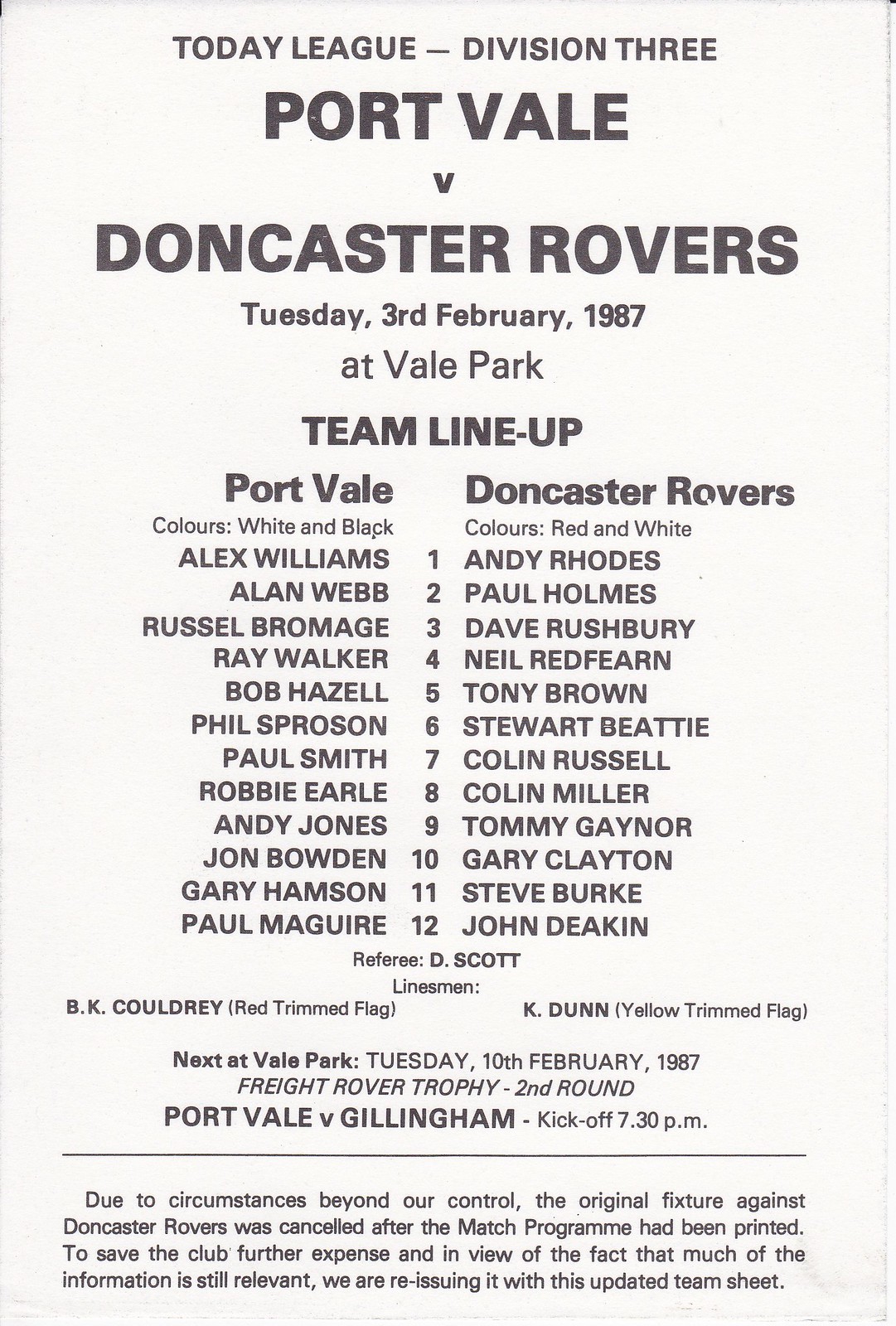This image appears to be a detailed page from a European football magazine, dated February 3rd, 1987. It outlines the lineup for a Division 3 match between Port Vale and Doncaster Rovers at Vale Park. The top of the page prominently features the match information: "Today League, Division 3, Port Vale v. Doncaster Rovers, Tuesday, 3rd February, 1987, at Vale Park, Team Lineup." Port Vale's lineup is listed on the left, with their team colors noted as white and black. Oppositely, Doncaster Rovers' lineup is listed on the right, with their team colors noted as red and white. Each lineup includes 12 player names.

Below the team lists, the officiating team is mentioned: Referee D. Scott, linesman B. K. Cauldry with a red-trimmed flag, and linesman K. Dunn with a yellow-trimmed flag. Additional information about the subsequent game is provided: "Port Vale v. Gillingham, kickoff 7.30pm."

At the bottom, a notice explains that the original fixture against Doncaster Rovers was canceled after the match program had been printed. To save costs and because much of the information remained relevant, the magazine was reissued with an updated team sheet.